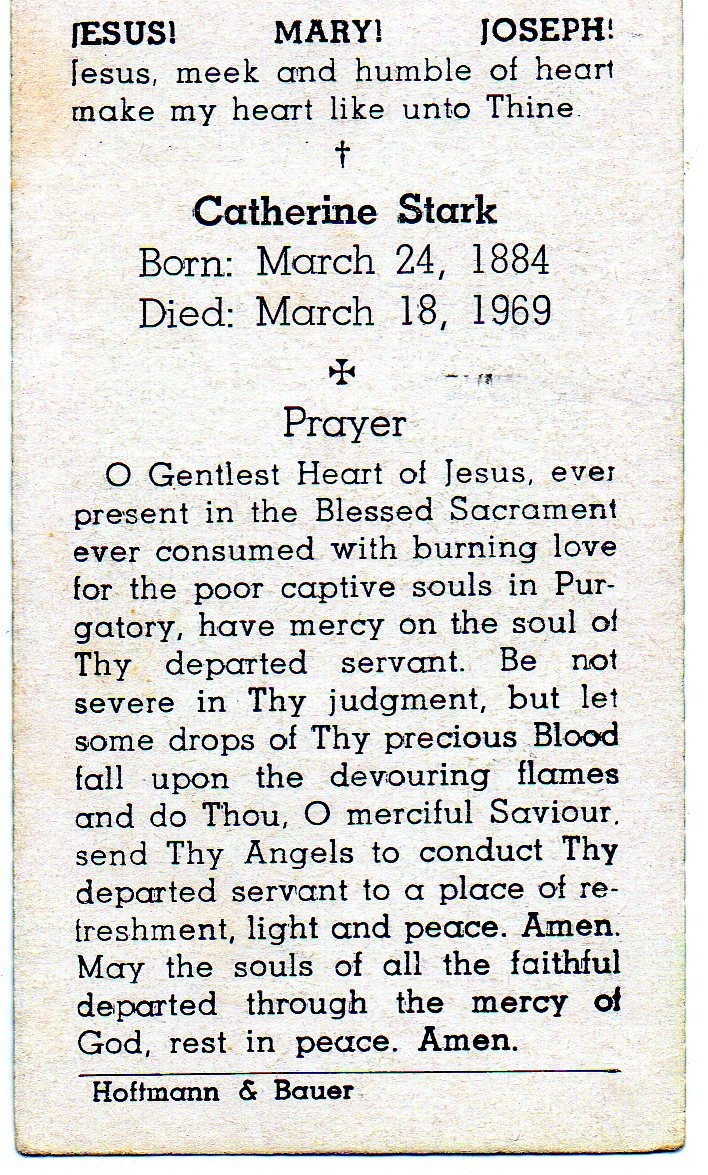This image depicts an old, light-tan memorial prayer card, likely handed out at a funeral or memorial service. At the very top, in bold black letters, it reads, "Jesus! Mary! Joseph!" followed by the invocation, "Jesus, meek and humble of heart, make my heart like unto thine." Below this, a small cross is displayed above the name, "Catherine Stark," who was born on March 24, 1884, and died on March 18, 1969. Another small iron cross follows, introducing a heartfelt prayer: "O gentlest heart of Jesus, ever present in the blessed sacrament, ever consumed with burning love for the poor captive souls in purgatory, have mercy on the soul of Thy departed servant. Be not severe in Thy judgment, but let some drops of Thy precious blood fall upon the devouring flames and do Thou, O merciful Savior, send Thy angels to conduct Thy departed servant to a place of refreshment, light, and peace. Amen. May the souls of the faithful departed, through the mercy of God, rest in peace. Amen." The card concludes with a line, beneath which the printer’s name, "Hoffman and Bauer," is inscribed on the bottom left.